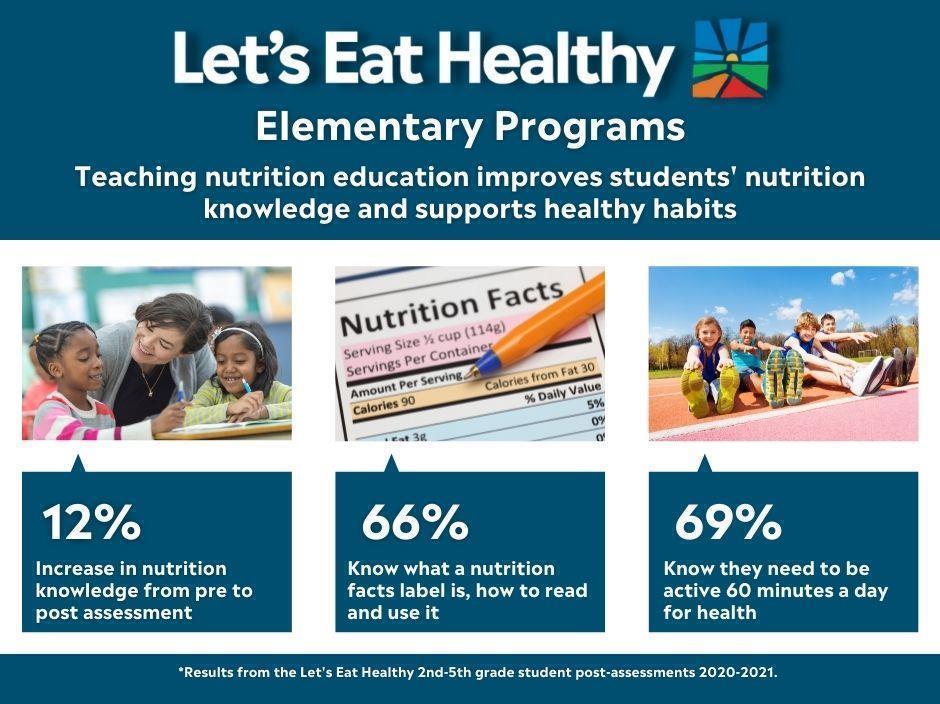The image is an informational poster titled "Let's Eat Healthy Elementary Programs," prominently displayed at the top on a blue background with large white letters. Adjacent to the title is a square emblem featuring a gradient of blue, yellow, green, orange, and red. Below the title, a series of statements emphasize the program's objectives: "Teaching Nutrition Education Improves Students' Nutrition Knowledge and Supports Healthy Habits." Three photographs are arranged horizontally beneath these words. The first image shows a woman in a blue shirt interacting with two children at a desk. The second image is a close-up of a nutrition label with an orange pen resting on it. The third image depicts children sitting on a track, displaying the soles of their colorful shoes. Below the images, blue rectangles with white text provide statistical results: "12% Increase in Nutrition Knowledge from Pre to Post Assessment," "66% Know What a Nutrition Facts Label Is, How to Read It and Use It," and "69% Know They Need to be Active for 60 Minutes a Day for Health." The poster concludes with a blue strip across the bottom, stating, "Results from Let's Eat Healthy 2nd to 5th Grade Student Post Assessments 2020-2021."